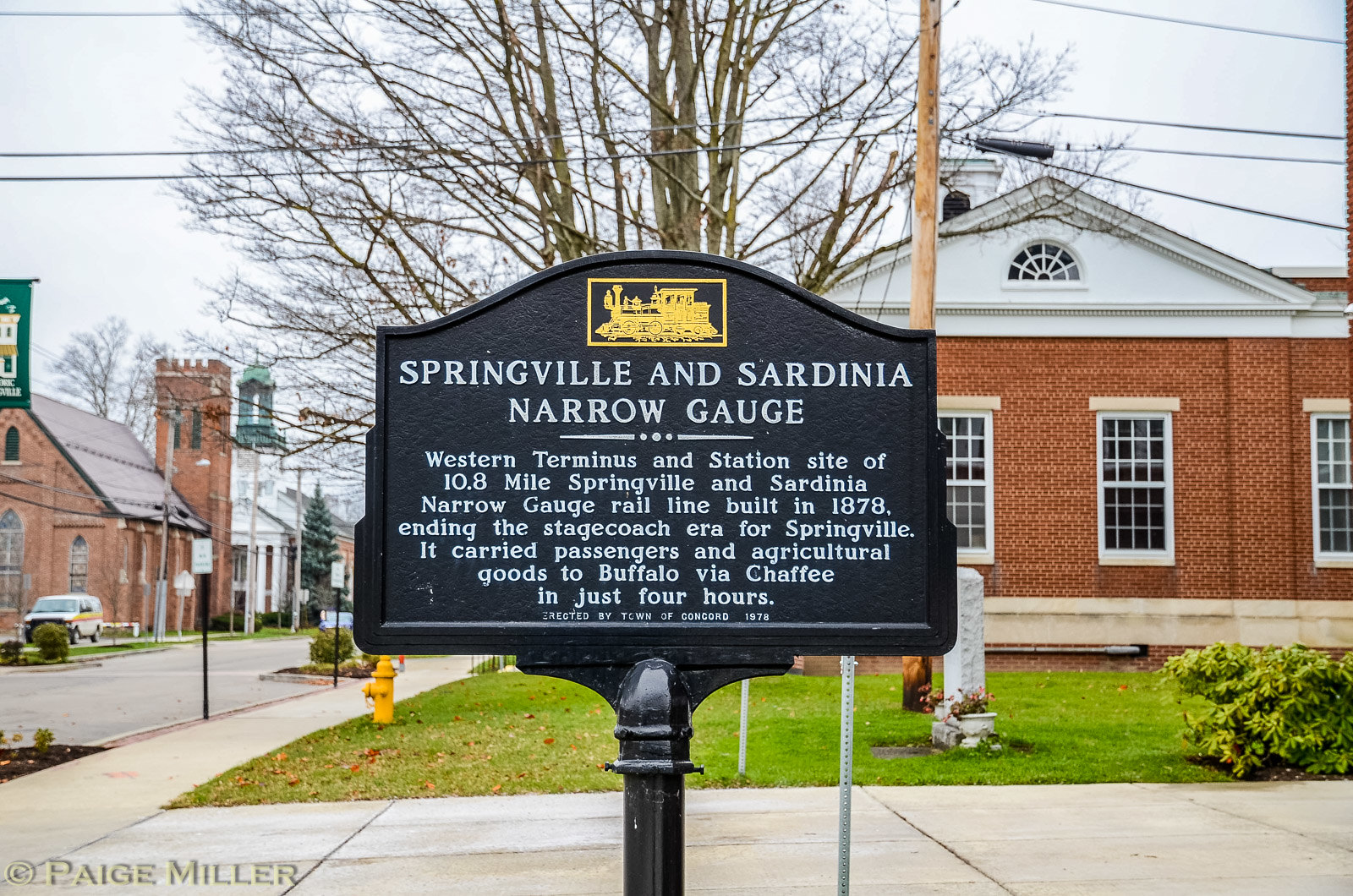The image captures a detailed historical plaque mounted on a black metal pole, displaying a rich narrative about the bygone era of rail travel. The plaque is a rectangular sign with a rounded top, featuring a drawing of a gold steam train engine and a gold rectangle against a black background. The main portion of the sign is black with white raised font, reading, "Springville and Sardinia Narrow Gauge. Western terminus and station site of the 10.8 mile Springville and Sardinia Narrow Gauge rail line built in 1878, ending the stagecoach era for Springville. It carried passengers and agricultural goods to Buffalo via Chaffee in just four hours. Erected by the Town of Concord 1978." The sign is situated outdoors, with the background revealing a townscape that includes red brick buildings, sidewalks, and a street to the left.